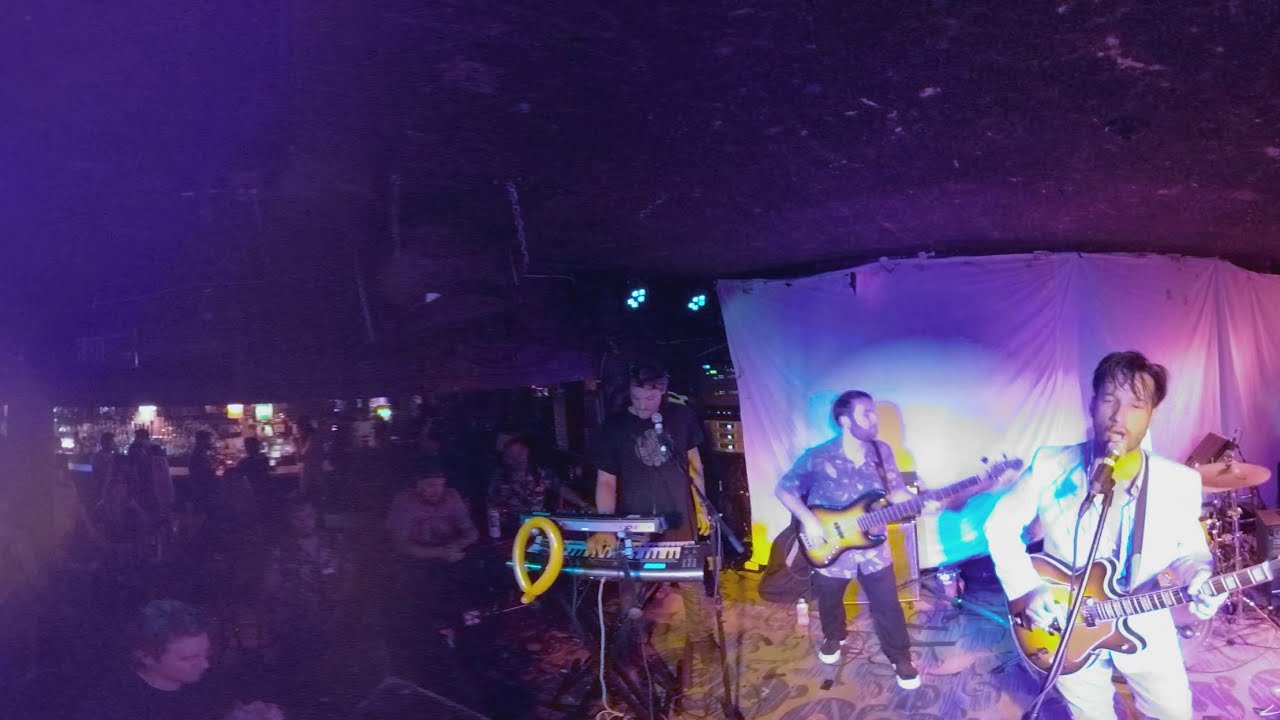The image depicts a live band performance in a dimly lit nightclub or dive bar, set in a horizontal rectangular frame. The background features a makeshift white sheet hung behind the band, casting a purple hue over the scene. On the left side, a small and casually dressed crowd can be seen sitting or standing, appearing rather unengaged and stared at the stage. The band consists of four members, each with dark hair. 

The lead singer, dressed in a white suit with a likely blue or white undershirt, plays a brown guitar and stands at the forefront. To his left, a man in a black t-shirt operates a silver keyboard marked with black and white keys, which has a light yellow balloon-like object attached to it. Another guitarist wearing a gray button-down shirt paired with dark pants and black and white shoes plays a guitar that is black on the edges with a yellow-orange center. Behind them, a drum set is partially visible, suggesting the presence of a drummer playing off-frame. The stage lighting includes various hues of purple, yellow, and blue from the ceiling fixtures, adding to the low-tech, lo-fi ambiance of the rock club. Despite the subdued energy of the audience, the band members appear intensely focused, with the lead singer exuding a rock star aura.